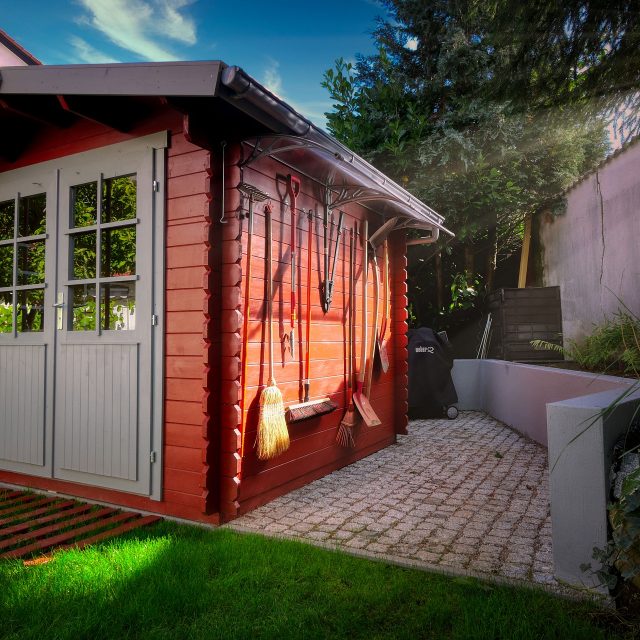This detailed snapshot captures a charming and well-organized backyard area. In the foreground, vibrant green grass leads the eye to a small, orangish-red garden shed with distinctive dual white front doors featuring faux window panes created by wooden overlays. Alongside the shed, a variety of garden tools, including brooms, head shears, a shovel, and a rake, are neatly mounted on the exterior wall under a protective overhang. The shed also has gray windows and doors framed by white trim descending from the roof.

Adjacent to the tool display runs a flagstone pathway with intermittent tufts of grass. This pathway is bordered by a short, white stucco retaining wall, beside which extends a taller wall that likely separates the yard from neighboring properties. A peaceful and functional stone patio area extends the usability of the space, adding both beauty and practicality.

In the background, a tall green tree reaches towards a blue sky dotted with clouds, while rays of sunshine spill over the walls, bathing the scene in a warm, inviting light. The presence of a discreet trash can and a painted red pallet in front of the shed's doors contribute to the area's utility, adding a touch of everyday realism to this idyllic backyard setting.